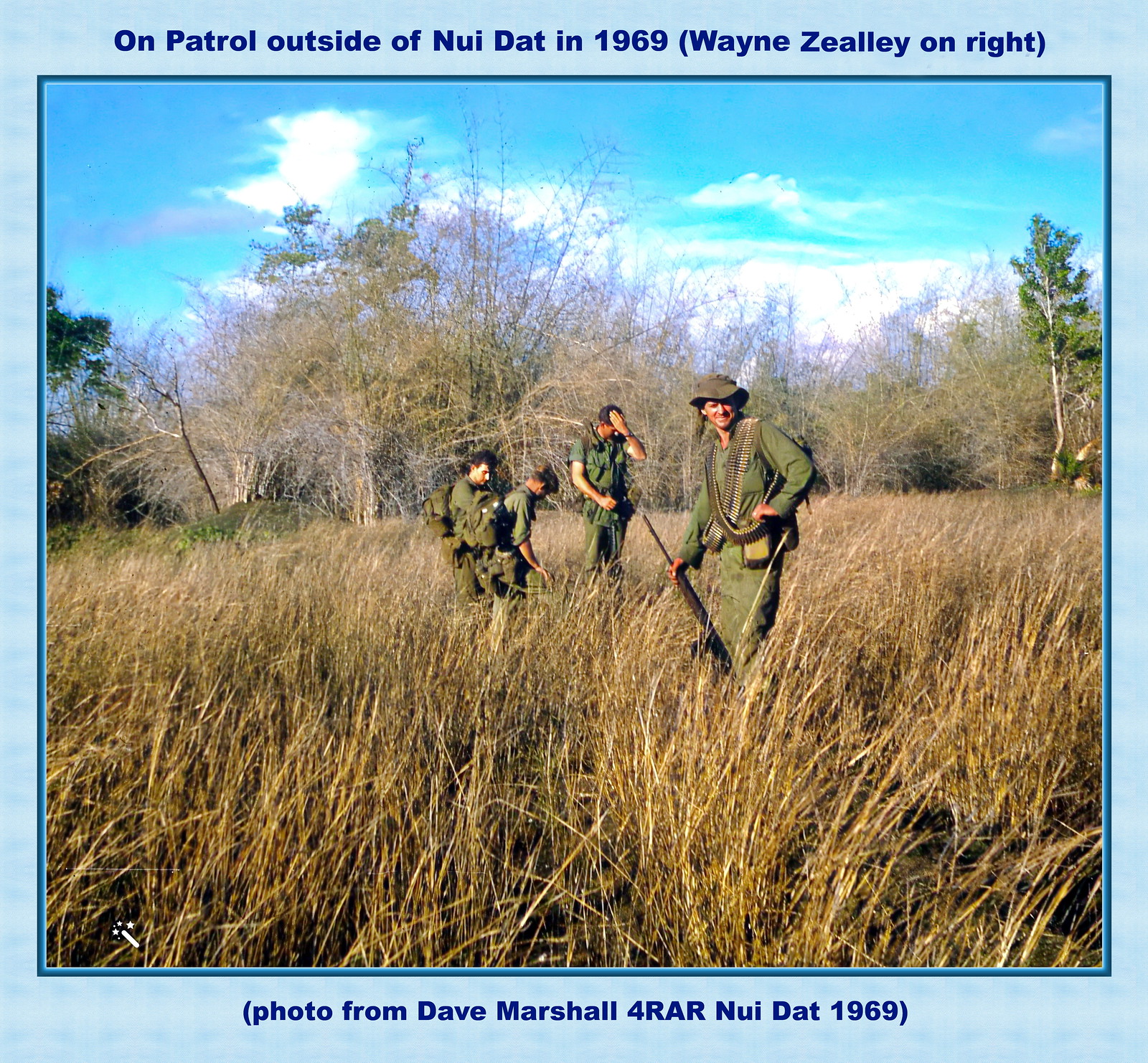This is a color photograph from 1969 featuring a group of four men in military fatigues, standing in a field of light brown grass. The photo has a light blue background with a blue square border. At the top, dark blue text reads "On patrol outside of New Dot in 1969" with "Wayne Zealy on right" in parentheses. The bottom text says, "Photo from Dave Marshall for RAR New Dot 1969" in parentheses. The men, possibly an American military unit during the Vietnam War, are positioned in front of scrubby brush and trees under a bright blue sky with white clouds. The man on the right is notable for wearing a bandolier of bullets over his shoulders, with a gun resting on the ground by his side.